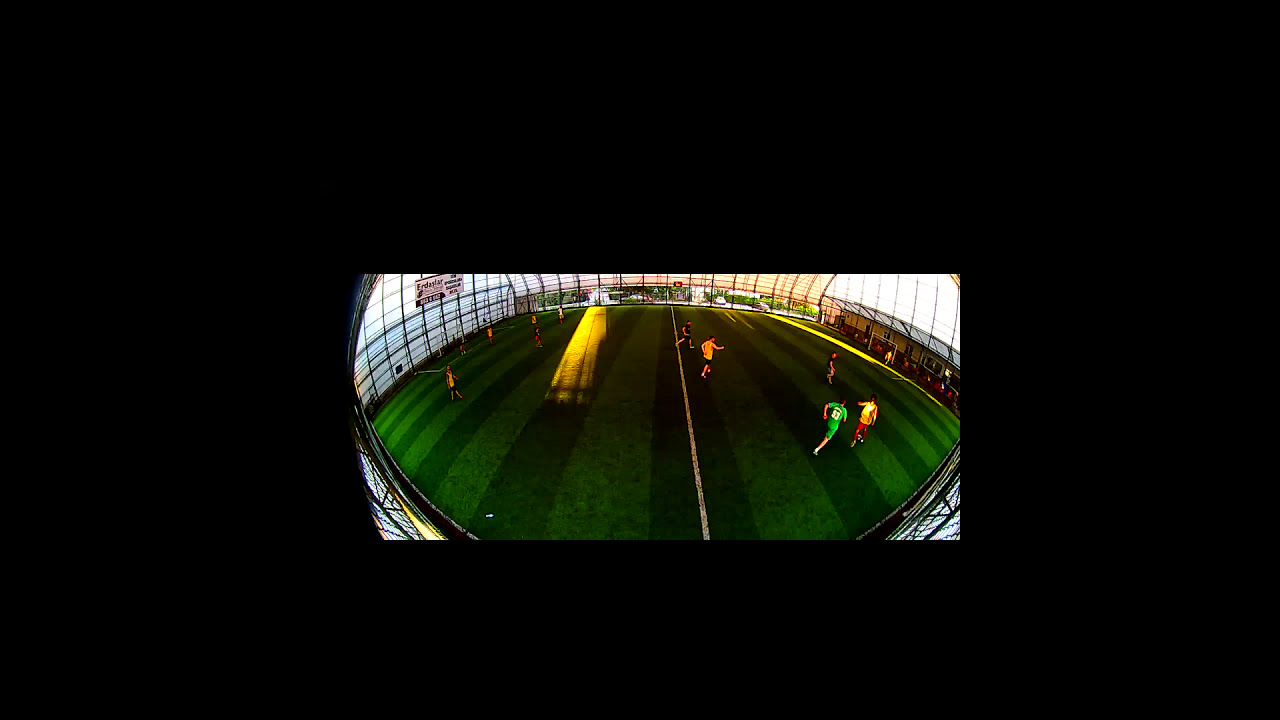The image depicts an indoor soccer game viewed through a fish-eye perspective. The grassy field shows alternating dark and light green vertical stripes, with a white line running down the middle. Players are dispersed across the field, wearing uniforms in various colors including green, yellow, red, and black. The stadium has a glass and metal frame, partially enclosed, with sunlight streaming through the glass, creating a yellow glare on the left side of the field towards the middle. The higher sections of the stadium, cut off from the image, suggest a large dome structure. On the sidelines, a few spectators can be seen, adding to the lively atmosphere of the match. The overall appearance of the image leans towards a cartoonish or video game-like style.